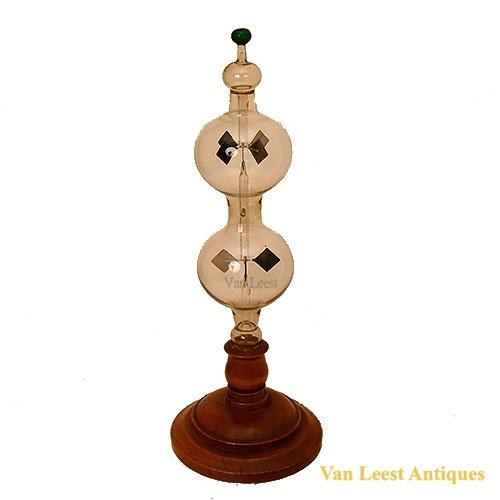The advertisement features a meticulously detailed image of an antique decorative object, set against a stark white background to highlight its intricacies. The centerpiece, likely a hand-blown glass sculpture or possibly lamp, stands out vividly. The object starts with an ornate wooden base, potentially a candle holder, transitioning into a slender stem that expands into a large, elegantly curved bulb. This bulb then narrows before broadening into a second bulb, which culminates in a smaller, circular top adorned with dark, diamond-like details. The overall coloration of the sculpture includes rich browns, ivories, and opaque blacks, contrasted by mustard yellow text. The text, "Van Leest Antiques," is prominently positioned at the bottom right, reinforcing the image's commercial intent for an antique store.